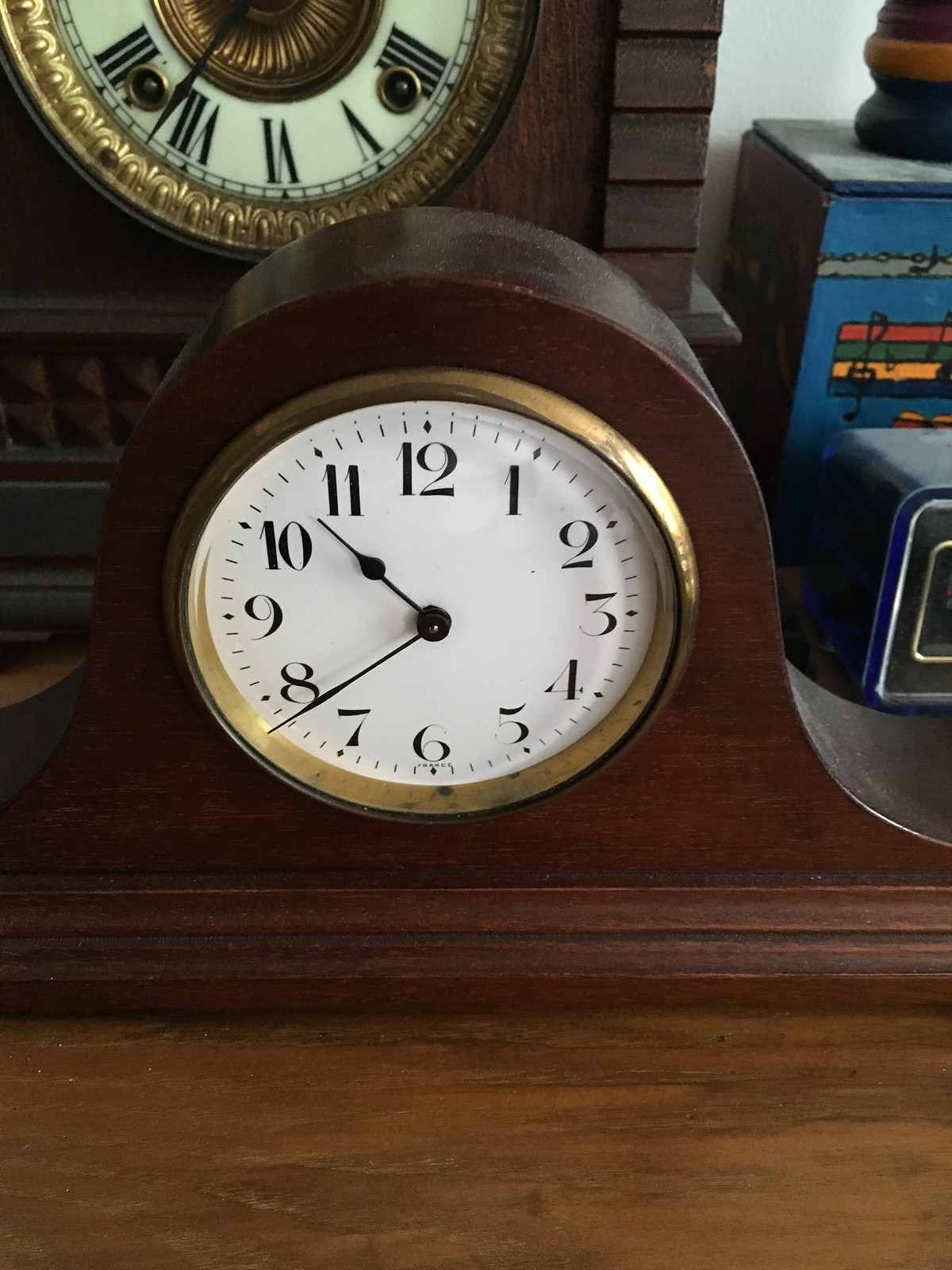In the image, prominently featured in the foreground, there is an analog clock with a dome shape and brown wooden frame, complete with bottom edges on both sides. The clock’s face is white, encased under glass, and circled by a golden trim. Black Arabic numerals from 1 to 12 mark the hours, with 12 at the top, 9 on the left, 3 on the right, and 6 on the bottom. The hour hand points between 10 and 11, while the minute hand sits between 7 and 8, indicating the time as 10:40. The clock is placed on a brown wooden table which has a bit of dust on its top edge. 

Adjacent to the right of the clock sits a blue object. Behind, there is a larger, ornate grandfather-style clock mounted on a darker brown wooden frame with intricate carvings. This clock also has a white face with a golden, ornate border and Roman numerals. It features two buttons at the front for key adjustment. This larger clock shares its space with a colorful cabinet featuring red, green, yellow, blue, and grey accents, complemented by a few other trinkets, including a colored box, on the lighter wooden shelf.